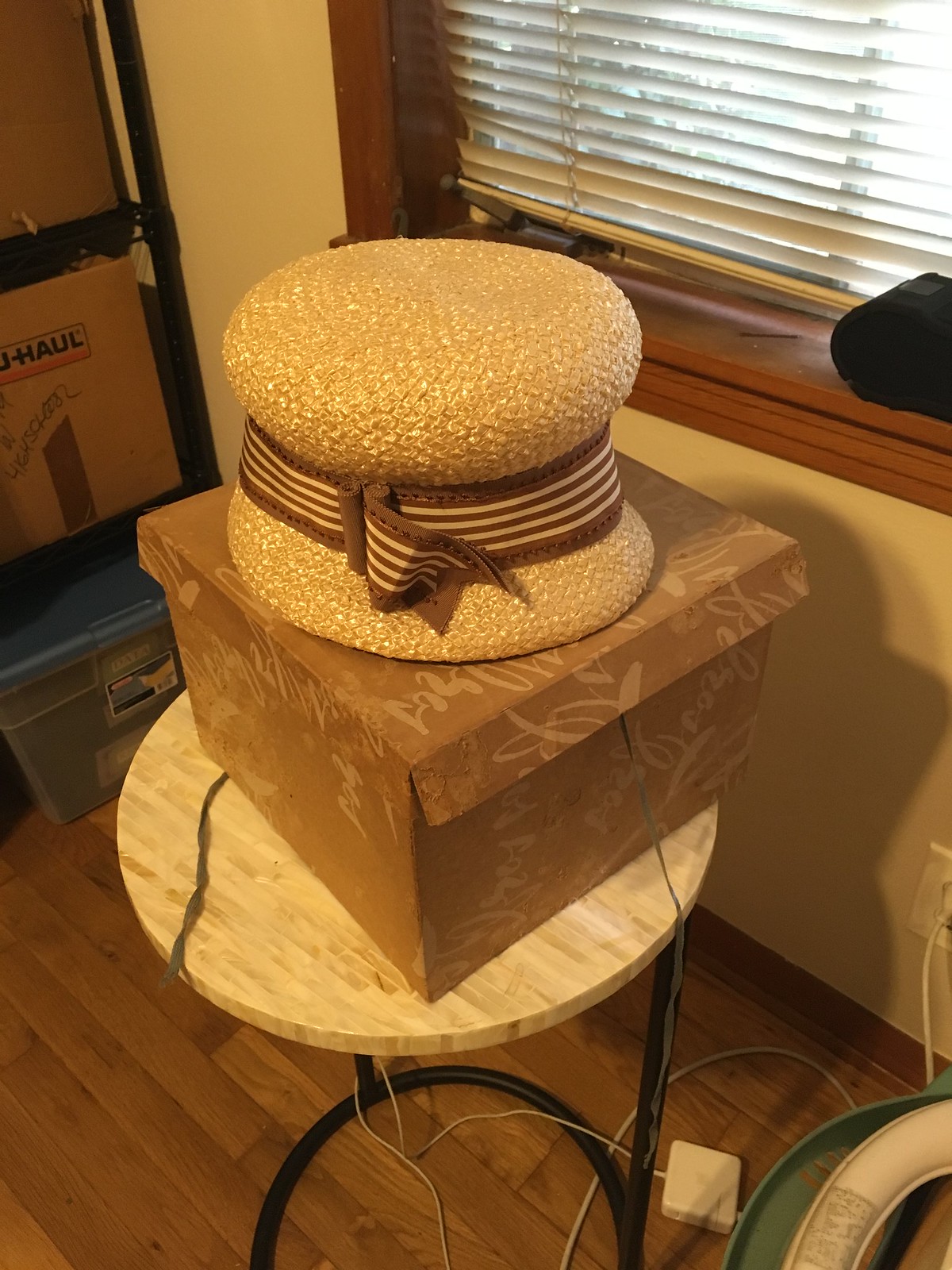This is a detailed color photograph taken inside someone's home, featuring a light brown, crinkly-textured hat sitting atop a matching brown hat box. The hat, a lady's design, is adorned with a brown and white striped ribbon around its center and has a tall, circular structure. The hat box, made of brown cardboard with beige and white decorative patterns, rests on a small, round marble-effect table, predominantly white with black legs leading to a round base. The table stands on a light brown wooden floor, complementing the shades of brown in the photograph. To the top right, a window with a dark wooden frame set in a cream-colored wall features closed horizontal blinds. In the top left corner, a shelving unit holds a plastic bin with a blue lid and various boxes. In the bottom right corner, a small plastic ring is visible on the floor.